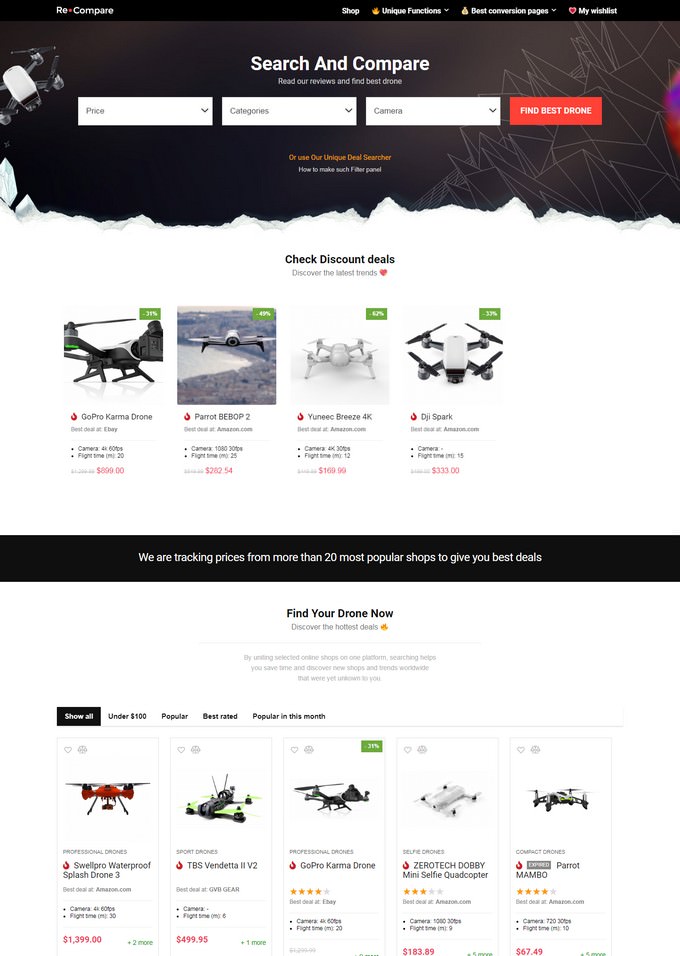The image is a portrait-oriented screenshot of a web page, with dimensions suggesting it is about twice as tall as it is wide. The topmost part of the page features a gray or black header, with some white text on the left that reads "Compare" (though the first word is unclear), and a series of white buttons. The first button is labeled "Shop," accompanied by three additional buttons with icons beside them.

Beneath this header is a black box with a white header that reads "Search and Compare" in white font. Within this section, there are three long, rectangular drop-down boxes side by side, each displaying different categories such as price and others that are too small to decipher. Adjacent to these boxes, there is a red search button with white text that says "Find Best Drone."

Further down, an orange text followed by some white font appears, though the text is illegible due to its small size. Directly below this, another black header reads "Check Discount Deals," showcasing four drone thumbnails. This is followed by a long, rectangular black box with white font.

The next section features another header, "Find Your Drone Now," with a search category area. The leftmost search category is highlighted in black, leading into a display of five drone thumbnails, each accompanied by relevant information beneath them.